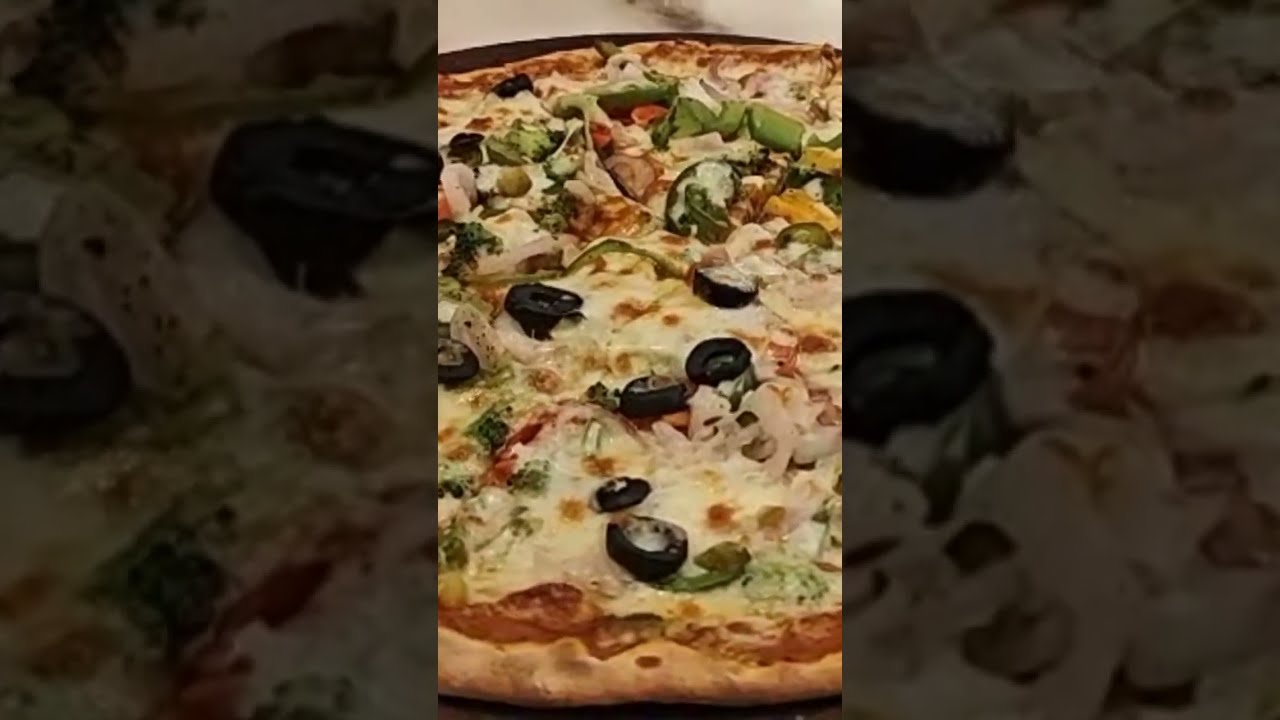This image shows a vertical strip of a supreme-style pizza with various toppings, centered within a horizontal rectangular frame that has dark, obscured sides. The pizza appears to be freshly baked and is still sitting in the pan. The toppings are diverse and include sliced black olives, onions, green peppers, mushrooms, and possibly pieces of broccoli. The pizza is covered with a generous amount of cheese, which is browned in certain areas from the hot oven, revealing patches of tomato sauce underneath. The image has a dated, yellowish tint, suggesting it might be from an old photograph or video with poor lighting. Some of the pizza appears to be cut, although this detail is not fully clear. The edges of the crust are visible, and the scene seems to be set on a whitish marble table.